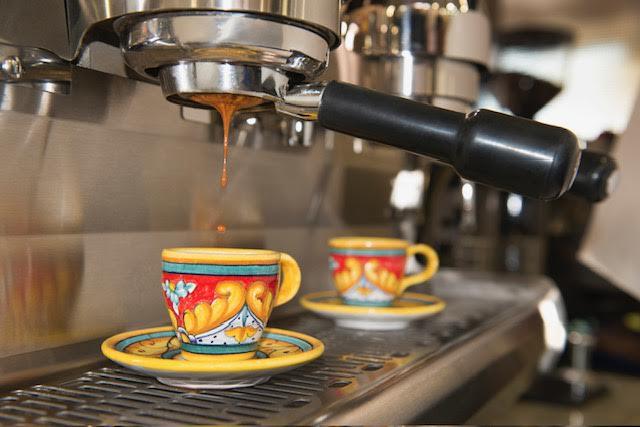This detailed photograph, likely taken behind the scenes at a restaurant or coffee shop, showcases a sleek, bright silver espresso machine mid-operation. The machine, which appears new and impeccably clean, features a prominent black handle and a grate beneath the cups to catch any spills. Positioned under the spout is an ornate ceramic cup, which is part of a matching set, awaiting drops of rich espresso. This cup, with its vivid yellow lid and handle, boasts an intricate Aztec-like design, incorporating hues of light blue and light red around its exterior, and sits on a coordinating yellow and green saucer. In the foreground, the sharp, bright colors of this cup and saucer contrast with the slightly blurred identical set in the background, which is waiting for its turn. The overall composition highlights the artistry and precision of coffee preparation, blending functionality with aesthetic appeal.